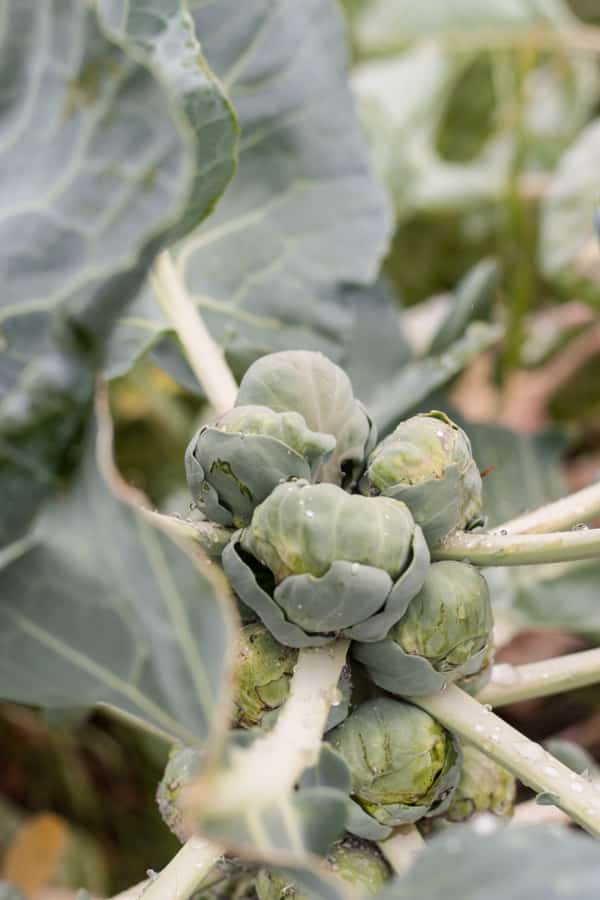The naturally taken photograph captures a close-up of a cabbage plant with light green stems radiating from a central point. At the center, there are several ball-shaped buds, which appear to be immature cabbages, tinged with green and yellow hues, and speckled with white spots. These buds are surrounded by large, dark green leaves that have light green veins running through them. The stems and stalks, which extend throughout the image, display short greenish thorns. The foreground plant stands out sharply against a blurred background filled with more green foliage. Rain has recently fallen, as evidenced by the water droplets visible on various parts of the plant, including the stems in the middle and at the bottom of the image. The lighting suggests an overcast sky, adding to the fresh, post-rain atmosphere of the scene.